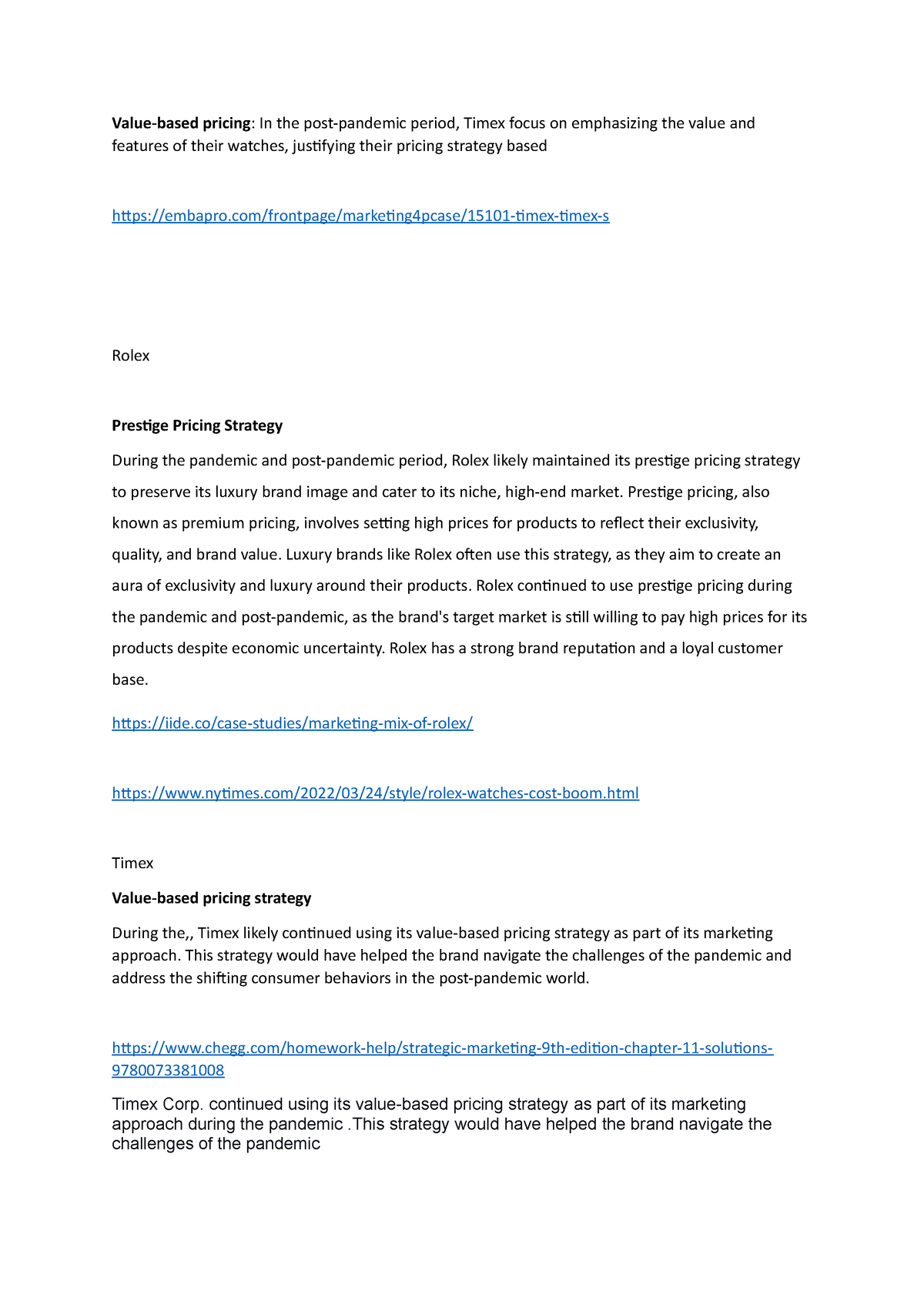An image captured from a cell phone screen displays a detailed analysis and comparison of pricing strategies by Timex and Rolex in the post-pandemic era. The header reads "Value-Based Pricing," followed by a paragraph describing Timex's focus on emphasizing the value and features of their watches to justify their pricing strategy post-pandemic. A clickable link titled "Timex Times" is included.

Further down, the text shifts to Rolex, introducing the concept of "Prestige Pricing Strategy." It explains how Rolex likely maintained its premium pricing strategy during and after the pandemic to preserve its luxury brand image and cater to its high-end market. Prestige pricing, also known as premium pricing, involves setting high prices to reflect a product's exclusivity, quality, and brand value. Luxury brands like Rolex use this strategy to create an aura of exclusivity and luxury around their products. The paragraph continues, indicating that Rolex's target market remains willing to pay high prices for its timepieces even during the pandemic and post-pandemic period.

Additionally, the page includes two more blue links and mentions Timex again, adding further details and links at the bottom.